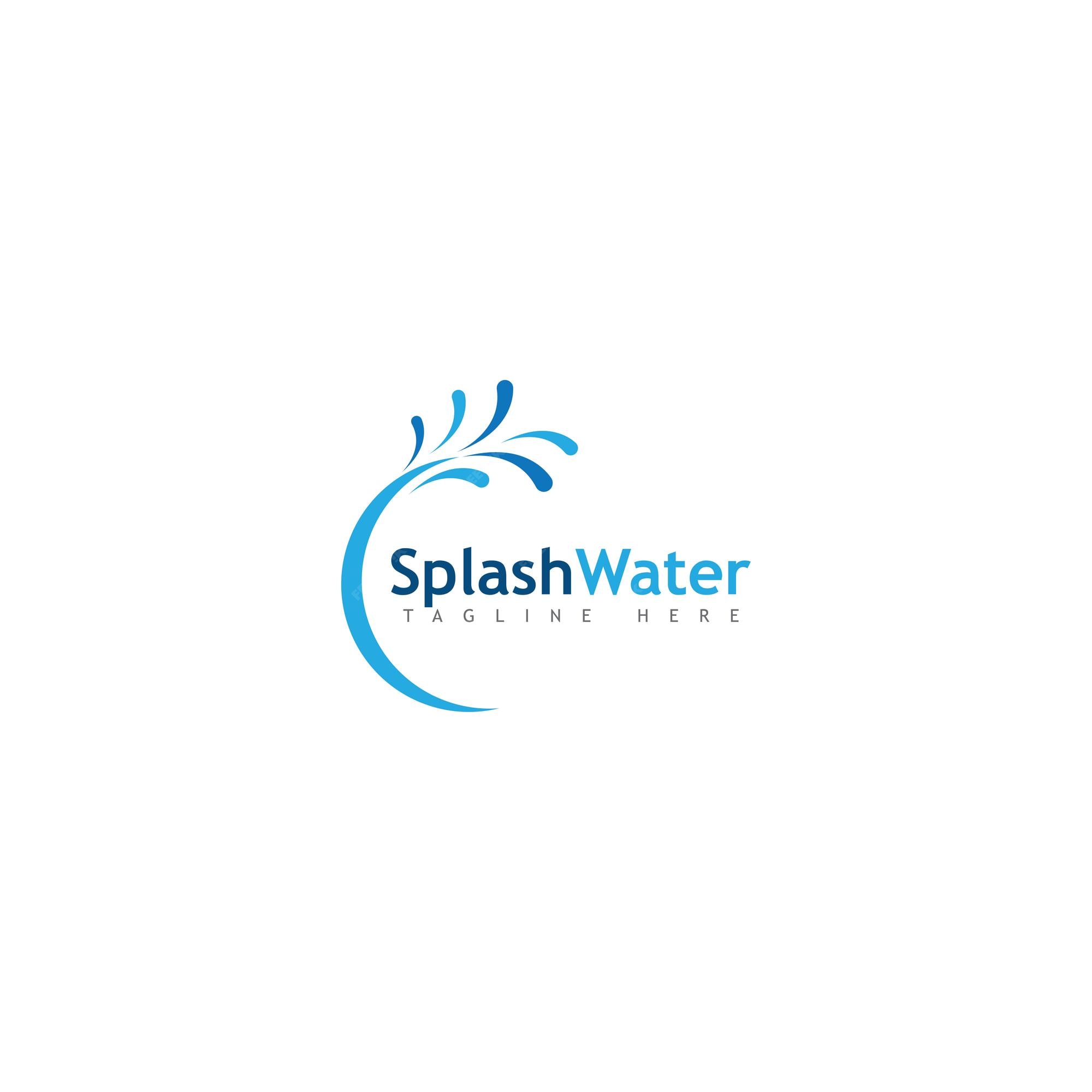The image features a simple yet striking logo for Splash Water, displayed against a white background. The logo prominently showcases the words "Splash Water" with "Splash" rendered in a dark blue font and "Water" in a lighter blue font. Beneath these words, the tagline "TAGLINE HERE" appears in small, all-caps black letters.

To the left of the text, there is a dynamic wave or tide shape, resembling a C or half-moon arc that swirls upwards and partially envelops the text. This wave is colored in a medium blue, and it is accentuated by several droplets of water that splash out from its crest, varying in shades from medium to dark blue. The overall design evokes the image of a vigorous water splash, as though someone had jumped into a pool, reinforcing the brand identity of Splash Water.